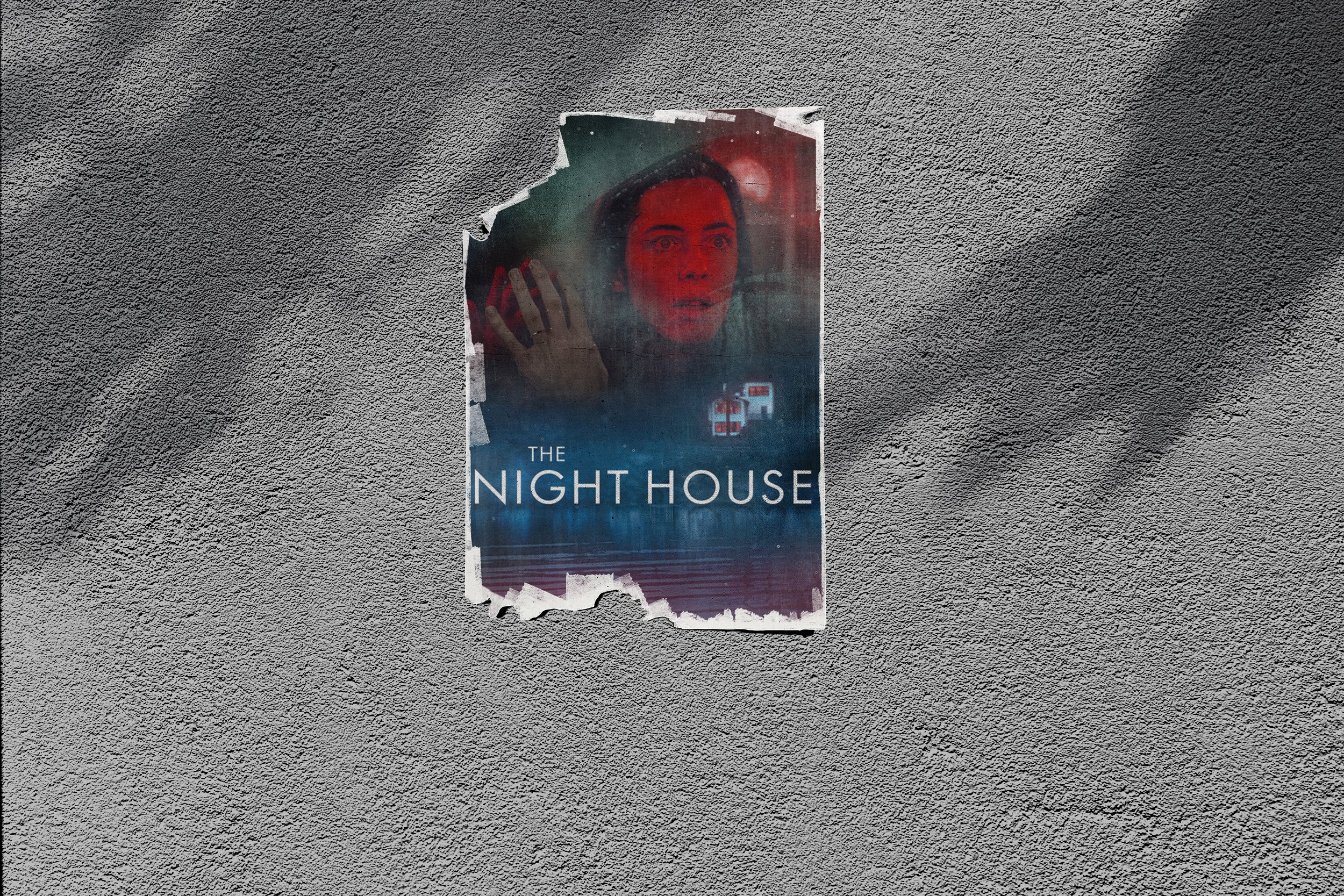The image displays a textured gray background, reminiscent of a stucco or concrete surface, with darker shadows resembling tree branches cast across it. At the center of this background is a ripped and jagged poster for a movie titled "The Night House." The poster appears deliberately torn, with the top left corner missing and chunks ripped out from the bottom left. 

Prominently featured on the poster is an eerie, red-tinted image of a woman's face, with her expression conveying alarm or shock. Her hand is raised as if she has just wiped condensation off a window or mirror. Below the image, the movie title "The Night House" is displayed in white text. The poster's overall color scheme includes deep blue, maroon, and greenish hues, adding to the dramatic and ominous feel, suggesting it is a horror movie. The woman's facial expression and the stylistic elements of the poster imply a narrative filled with suspense and fear.

Additionally, there is a small detail of a for-sale sign, which could hint at an intriguing plot point in the movie. Overall, the setting and the design of the poster create a visually compelling and suspenseful atmosphere.